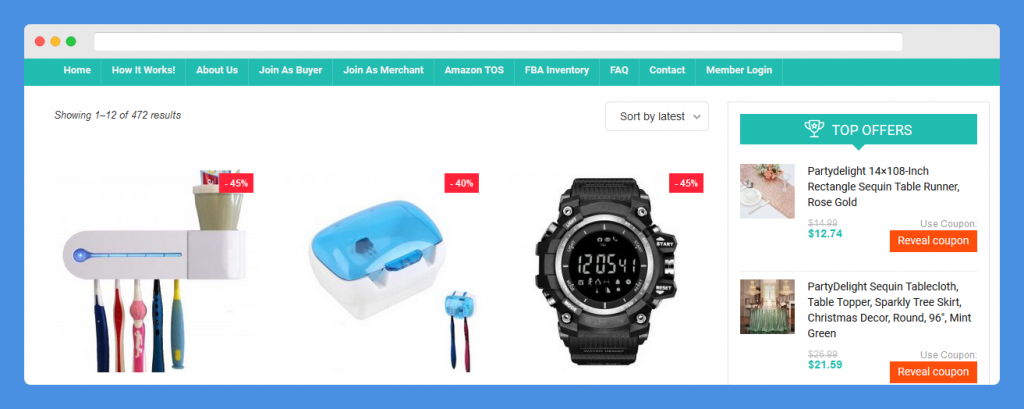This vibrant and colorful website features a distinct blue border on the top, bottom, and sides, while the interior background is primarily white with a touch of gray near the search bar. A prominent green strip at the top provides navigation options, including: Home, How It Works, About Us, Join as Buyer, Join as Merchant, Amazon TO3 or TOB, FBA Inventory, FAQ, Contact, and Member Login.

The visual content on the page is diverse and eye-catching. The first image showcases a variety of toothbrushes in shades of pink, white, and blue, neatly hanging, with a cup positioned atop the toothbrush holder. The following image displays a footbath featuring a white bottom and blue top. Afterward, there's a separate image of a toothbrush holder followed by an image of a men’s watch displaying the time 12:05, characterized by its chunky and robust design.

On the right side of the page under the "Top Offers" section, there are promotional items listed, including a Party Lights, a Party Delights Rectangle Sequins Table Runner, and a Party Delights Sequin Tablecloth Table Topper. This detailed layout highlights the varied merchandise and structured navigation options available on the website.